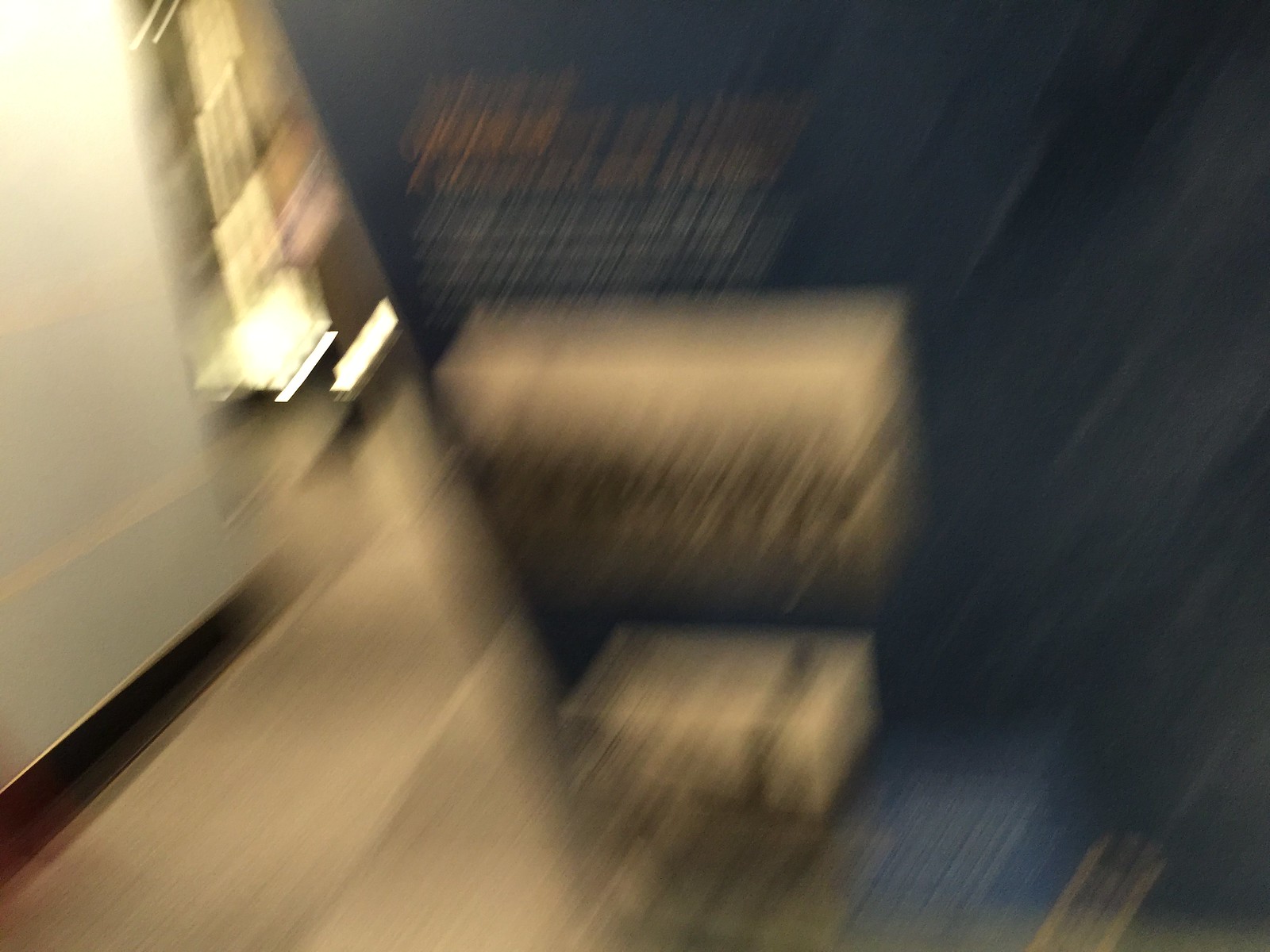This extremely blurry and out-of-focus image is difficult to discern, but several elements are vaguely identifiable. The left side of the image seems to depict a light-colored hallway, possibly inside a home, with white walls and brown wainscoting leading into a smooth beige-colored wooden floor. The background appears to contain streaks of light and alternating beige and brown squares. Centrally located in the foreground, there appear to be two Amazon packages—one smaller box with a vertically oriented black strip and a larger box with a horizontally oriented black strip. The right side of the image is much darker, featuring a bluish-black background with an indistinct promotional board or picture board that has some orange and white text at the top left corner. However, the lack of focus renders the text unreadable and the overall scene very hard to discern.